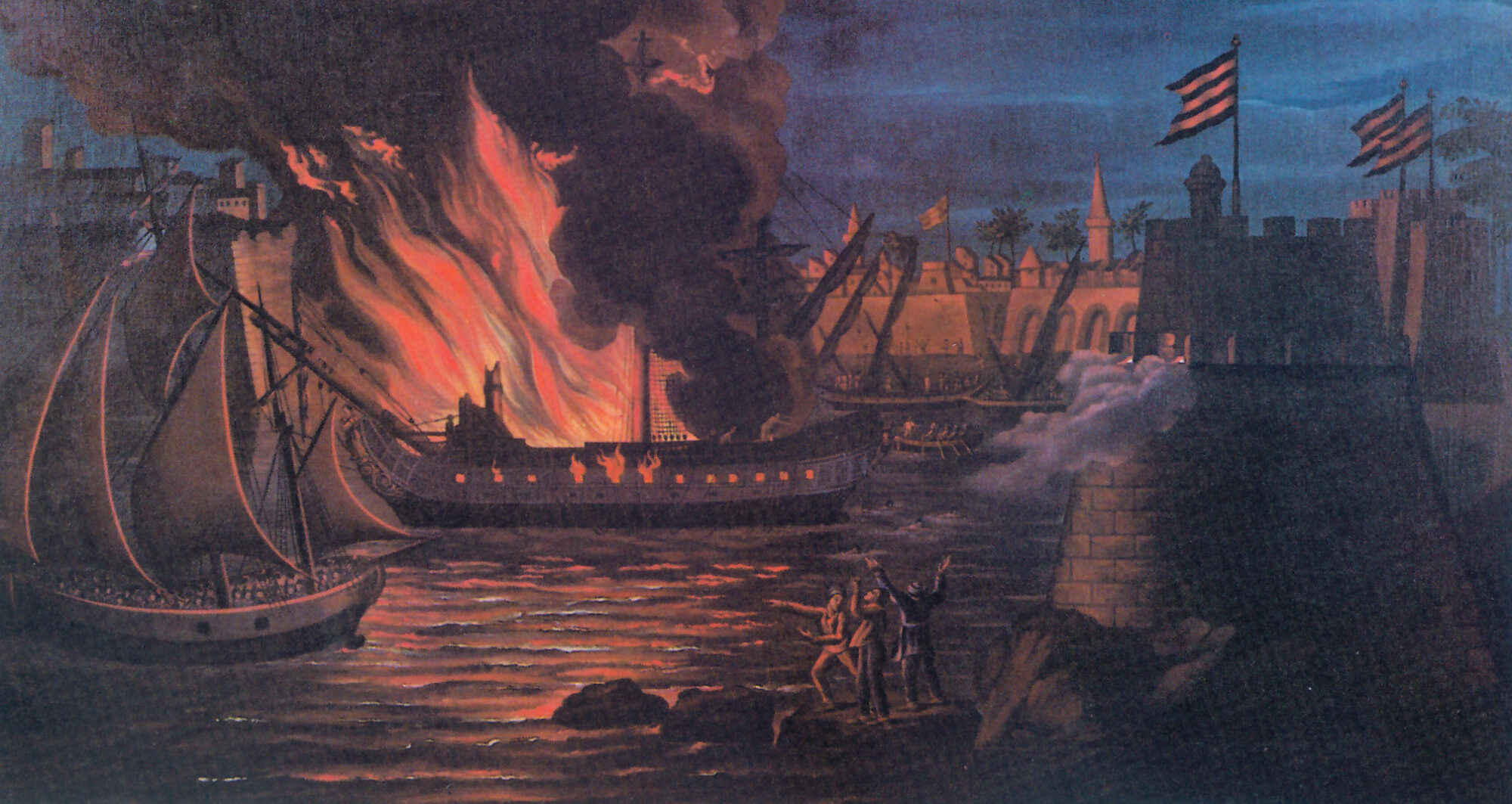This evocative painting captures a dramatic nighttime scene at a colonial-era port, under the ominous glow of fire and the tranquil blue of the evening sky. Dominating the composition, a large ship fiercely burns in the water, its mast partially collapsed and enveloped in towering flames and billowing smoke. Nearby, another vessel with three sails remains afloat, casting a stark contrast against the inferno. The port is fortified by castle-topped structures, adorned with three tattered flags that appear either black and white or blue and white striped, all fluttering towards the sea. In the bottom center, three figures stand on a rock, gesturing animatedly towards the spectacle before them, accentuating the sense of urgency and chaos. The surrounding buildings and fortifications suggest the presence of a military base. The overall palette is a mix of dark hues, punctuated intensely by the reds and oranges of the flames, amplifying the scene’s dramatic intensity.